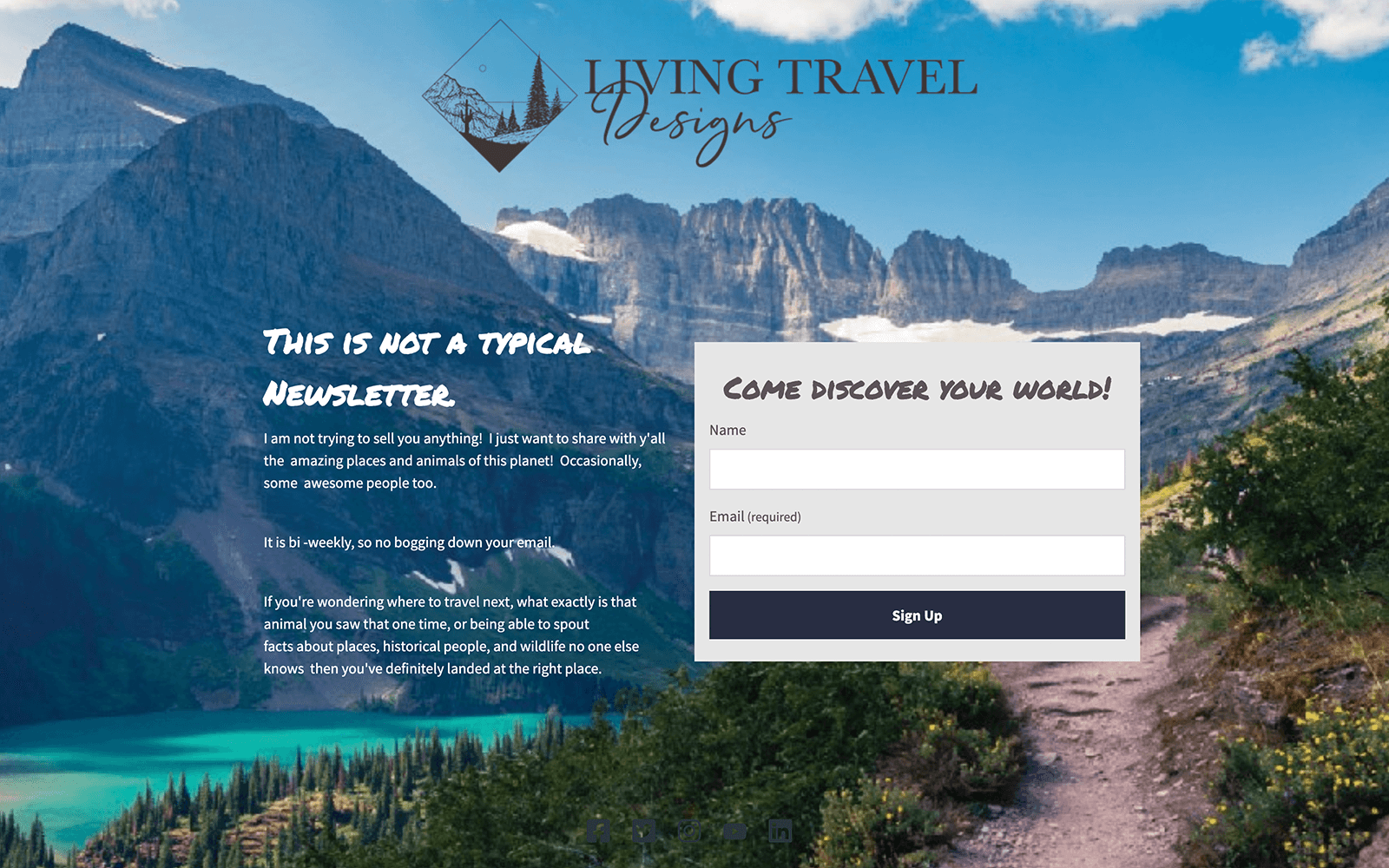**Descriptive Caption:**

A captivating screenshot of a travel website is presented, showcasing a breathtaking backdrop of a mountain range with a hiking path meandering up a lush, grassy hillside. The path overlooks a serene lake that nestles between the hillside and the distant mountains. The sky above is a clear blue, adorned with a few fluffy white clouds. Emblazoned across the sky area is a diamond-shaped logo featuring stylized mountains and trees, next to the bold text "Living Travel Designs."

The main content of the website is divided into two sections. On the left side, a headline reads, "This is Not a Typical Newsletter," accompanied by a brief description underneath. On the right side, an enticing call-to-action, "Come Discover Your World," introduces an input form comprised of text fields for a visitor's name and email address, along with a rectangular, light gray sign-up button bearing black text.

The entire layout of the website reflects an invitation to adventure and exploration, tailored for wanderlust-driven visitors eager to stay connected with travel inspirations and updates.